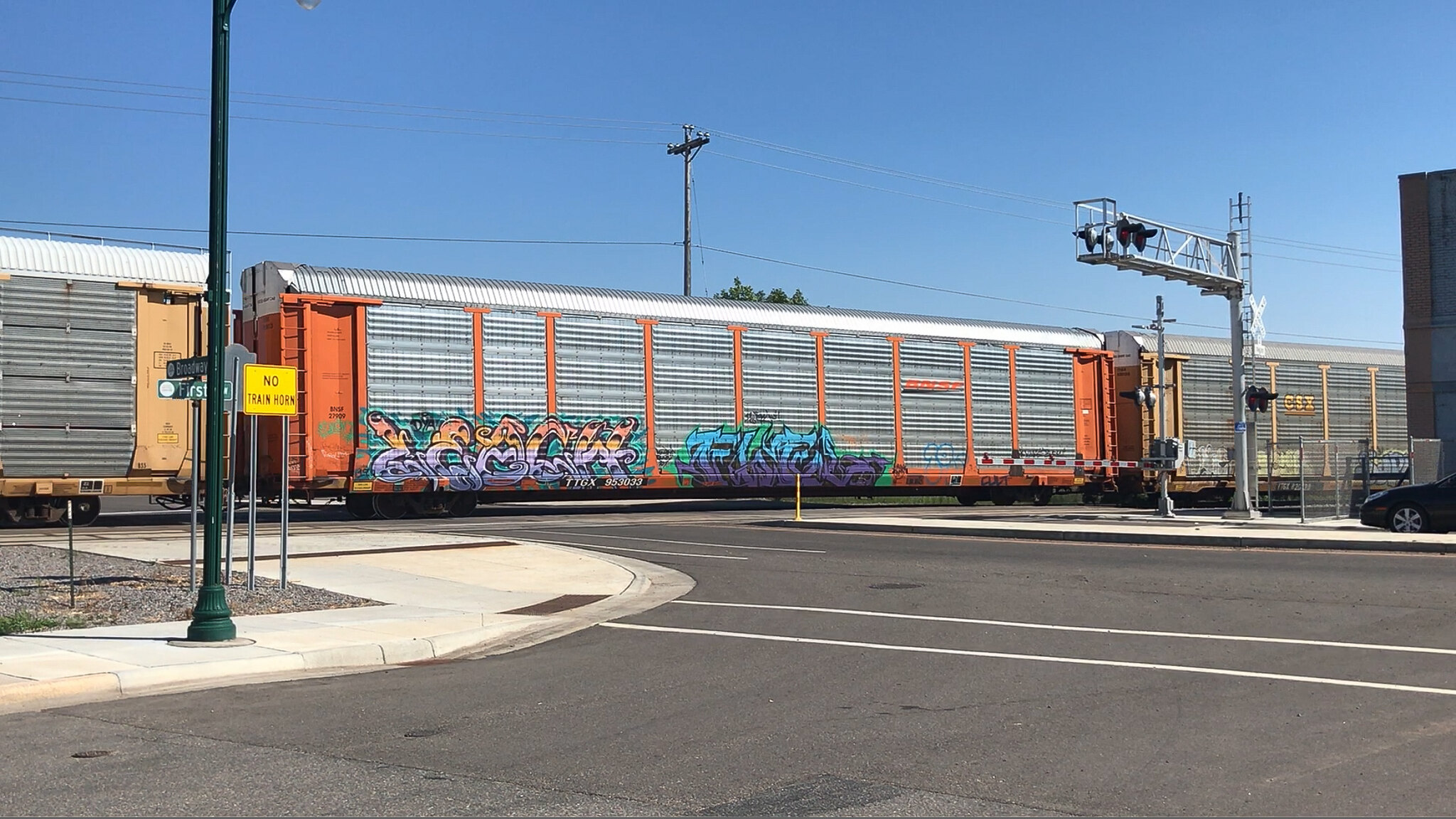The image presents a diagonally cropped color photograph capturing a train stopped at an intersection under a sunny sky. The focal point is an orange railcar adorned with graffiti, including the words "Escu" and "Fuego", positioned centrally between two other railcars. The railcar to the left is a light beige-orange, while the one to the right is a golden yellow, both topped with silver. The scene occurs in the middle of the day, revealing a paved road with a vehicle intersection just before the railroad tracks, accompanied by sidewalks and a tall green light pole on the left. The metal grating of the train crossing apparatus is visible on the right-hand side, emphasizing the intersection's functionality and the urban environment.